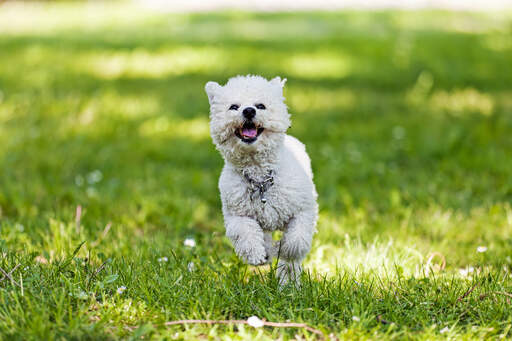In this vibrant outdoor photograph, a little white dog with fluffy, puffy fur is captured mid-run across a sun-dappled field of rich green grass. The dog, positioned centrally in the image, appears to be joyfully bounding towards the camera with its front paws raised and head slightly leaning to the left. Its mouth is open, revealing a pink tongue, and you can clearly see its expressive black eyes and nose. The dog wears a silver collar that catches the sunlight, adding a touch of brightness. The grassy field, dotted with a few daisies and sticks, is bathed in sunlight, creating patches of yellowish-green where the light breaks through the trees, even though the trees themselves are not visible. The entire scene takes place under a clear, sunny sky, emphasizing the lively and cheerful atmosphere of the image, which is slightly wider than it is tall.